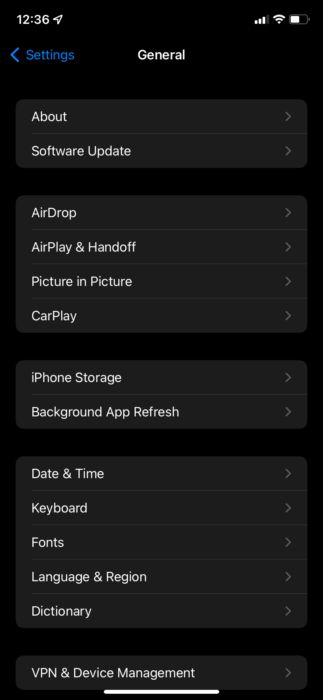The image depicts a screenshot of a cell phone displaying its "Settings" menu on a black background. At the top left corner, the time reads 12:36. The top right corner shows three signal bars, a full Wi-Fi symbol, and a half-full battery icon. Directly beneath this status bar, "Settings" is written in blue with a blue arrow beside it.

The main section of the screen displays the "General" settings. Listed below "General" are the following options, each boxed and separated by spaces:

1. **About**
2. **Software Update**

Another section follows, listing additional settings within boxes:

3. **AirDrop**
4. **AirPlay & Handoff**
5. **Picture in Picture**
6. **CarPlay**

Further down, another section presents more options:

7. **iPhone Storage**
8. **Background App Refresh**

Continuing downward, the settings list includes:

9. **Date & Time**
10. **Keyboard**
11. **Fonts**
12. **Language & Region**
13. **Dictionary**

At the very bottom of the screen, the final setting listed is:

14. **VPN & Device Management**

Each section is clearly delineated by spaces, making it easy to navigate through the different settings categories.